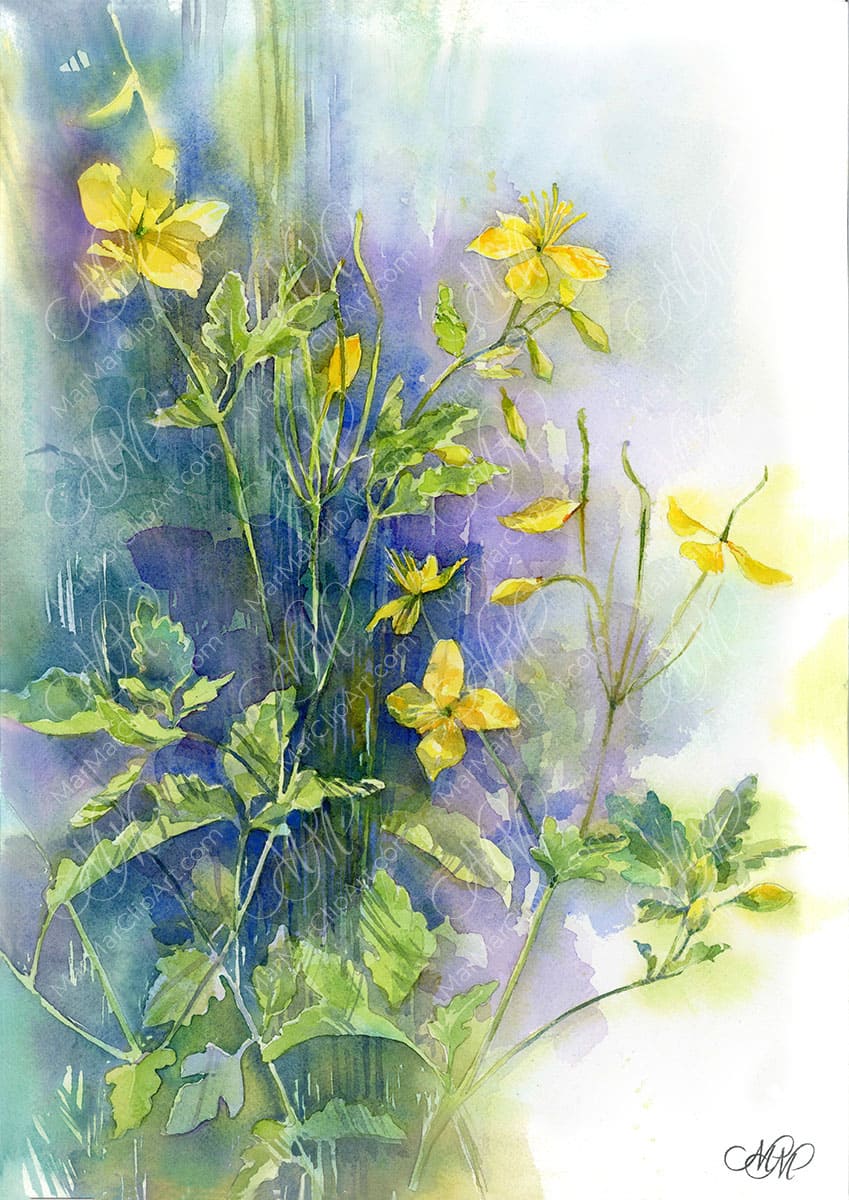The image is a detailed and artistic rendering of a plant featuring multiple green stalks extending upward into delicate yellow flowers, each with three to five petals. These flowers are accented by stringy structures at their centers and are surrounded by medium green leaves. The painting's background transitions from a richer blue and purple on the left, sprinkled with green streaks suggesting additional upright stalks, to a fully white background on the right. The composition includes several flower buds at various stages, with the central focal point being four prominent flowers—two at the top and two to the right. The plant stems and leaves spread vertically, with two to three main stems branching out and supporting buds and flowers. The bottom right corner of the artwork is marked with the initials "MM" in elegant calligraphy, adding a personal touch to this intricate watercolor painting.